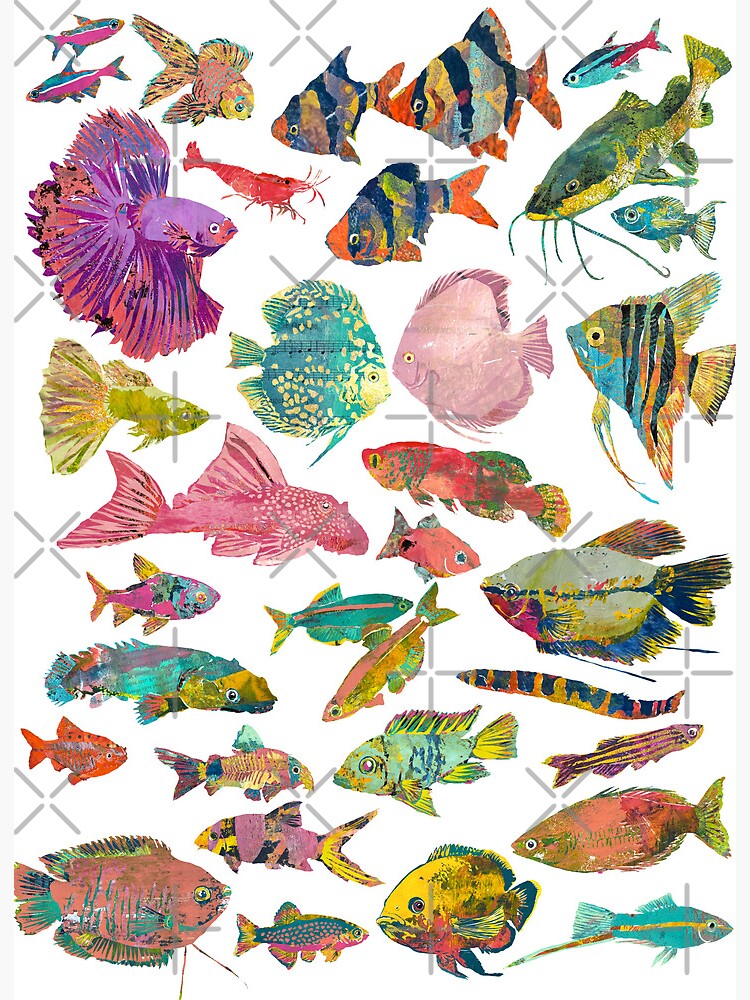The image features an intricate and dense assembly of various marine life illustrations, most of which appear to be computer-generated or potentially painted. On a vertically oriented, rectangular white background, numerous vibrant fish and a few crustaceans, including an eel-like creature and a shrimp or prawn, are clustered closely together. Scattered across the paper are light gray X shapes, likely serving as a watermark or copyright protection.

The fish are depicted in a rainbow of pastel colors, with predominant hues of pink, purple, blue, and touches of yellow, creating a visually striking and dynamic composition. Each fish showcases unique characteristics: some fish resemble goldfish, sunfish, and clownfish, while others appear similar to catfish with their distinctive whiskers. The collection also includes tropical species and variations in size, shape, and pattern, such as betta fish with their flamboyant fins and striped fish with transverse or longitudinal patterns.

Altogether, there are around 50 fish facing different directions—left, right, up, down—suggesting a sense of movement and liveliness within the static image. The meticulous detail in the patterns, gill types, and vibrant coloration underscores the diversity of species portrayed in this elaborate marine collage.